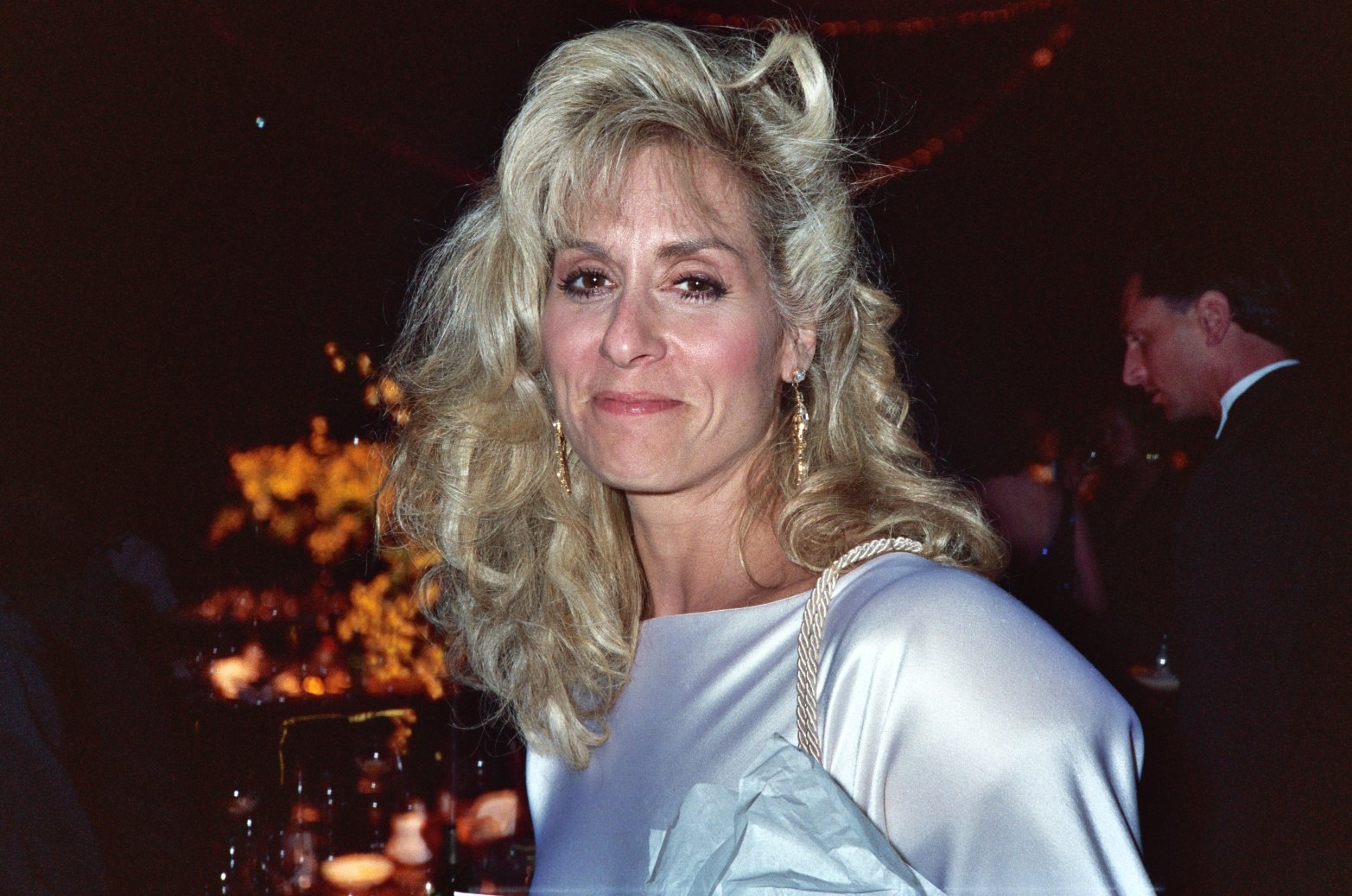The photo is an older, vintage-looking snapshot that appears to have been taken many years ago, reminiscent of something you might find in an old photo album. The setting is dimly lit, likely a party or a restaurant, with an overall dark and blurry background. 

In the foreground, there's a woman with light-skinned complexion and dirty blonde hair that is slightly messy and extends beyond her shoulders. She is smiling toward the camera, wearing a shiny bluish-white top and long, dangly earrings. A distinctive feature is her blue handbag, which has a gold rope handle and is draped over her shoulder.

In the background, partially obscured by the darkness, there's a gentleman in a dark suit jacket and a white collared shirt. He appears to be talking to someone and is seen from the side. Other indistinct shapes of people can be noticed, but they are not clearly visible. The background also includes some warm light sources—possibly candles or reflections—that add to the dim ambiance of the scene. The overall image is slightly blurry, contributing to its nostalgic feel.